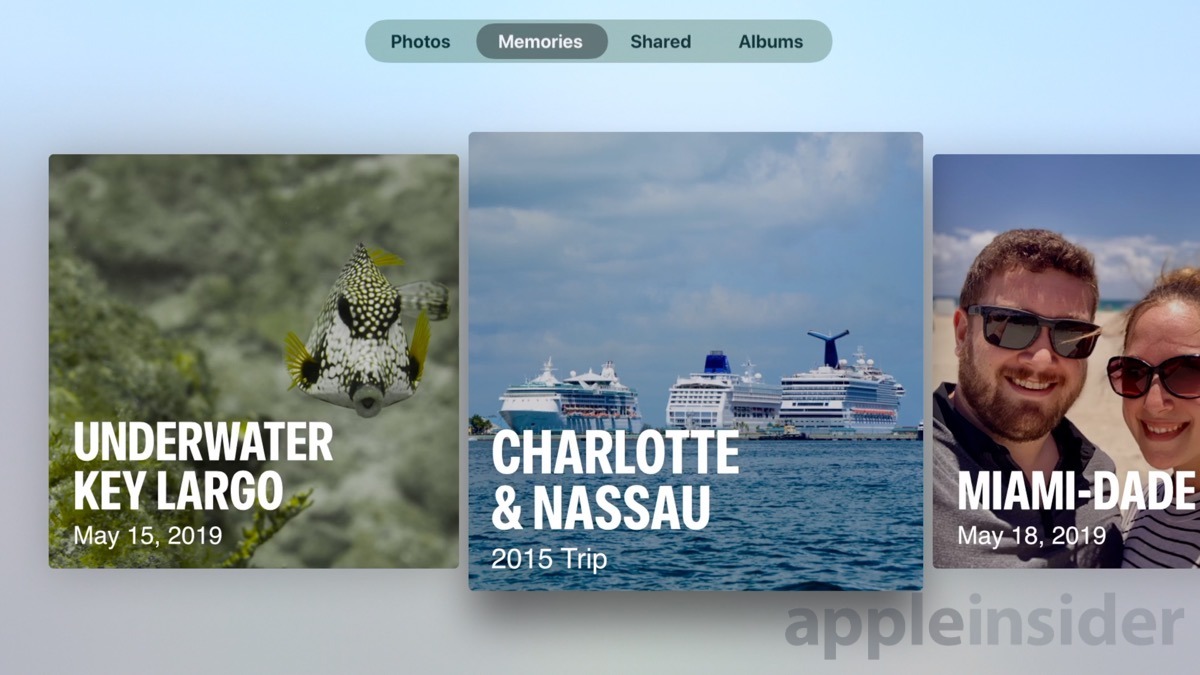Screenshot from Apple Insider: At the top of the website, there is a light blue bar with a gray circle in the middle, showcasing navigation options like "Photos," "Memories," "Shared," and "Albums." The "Memories" tab is currently selected. 

Below this bar, three images are displayed in a row:

1. **Underwater Key Largo, May 15th, 2019**: This image features a stunning underwater scene. A fish, identifiable by its unique coloring—black on top of the head with white polka dots, a predominantly white body with some black markings, and yellow fins—swims gracefully in the ocean.

2. **Charlotte and Nassau 2015 Trip**: This image captures a picturesque view of the ocean under a blue sky dotted with clouds. Centered in the scene are three large, white cruise ships.

3. **Miami Dade, May 18th, 2019**: This beach photograph shows a man and a woman enjoying their time in the sun. The man, positioned on the left, has brown hair, a mustache, a beard, and wears sunglasses and a gray shirt. The woman, on the right, also sports sunglasses and a gray and black striped shirt. Both are smiling, standing against the backdrop of a sandy beach and a blue sky with clouds.